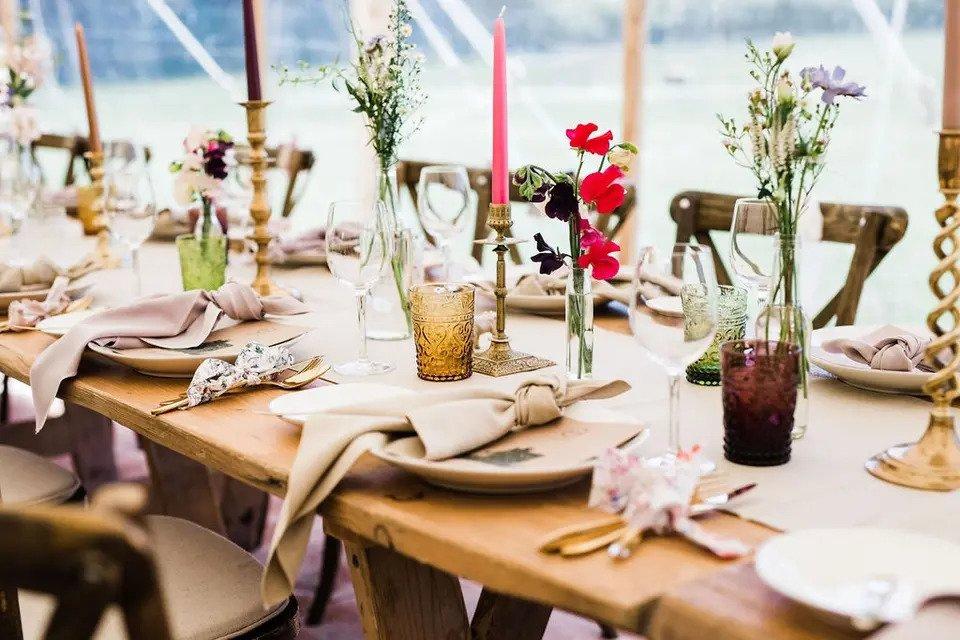This photograph captures an exquisitely arranged dinner table, likely situated in an upscale restaurant or a sophisticated home setting. The table itself is a light wooden live-edge piece, showcasing a rustic yet elegant grain. Each place setting includes white plates adorned with intricately knotted linen-colored napkins, paired with metallic or gold-colored utensils tied together with fabric knots in patterns of white and black spots or white and pink flowers. The multi-colored glass tumblers add a vibrant touch, with shades of green, yellow, red, dark blue, purple, and amber, complemented by clear glass wine glasses.

The centerpiece features a diverse arrangement of floral displays, using bottles and thin glass boxes filled with water to hold the stems. The flowers themselves are a mix of colors including red and white, adding to the visual appeal. The table is further decorated with a variety of candles that alternate in height and color, with some brown and others pink, casting a warm, inviting glow over the entire setting. The seats, draped in fabric, surround the table, completing the lavish and meticulously detailed dining scene.